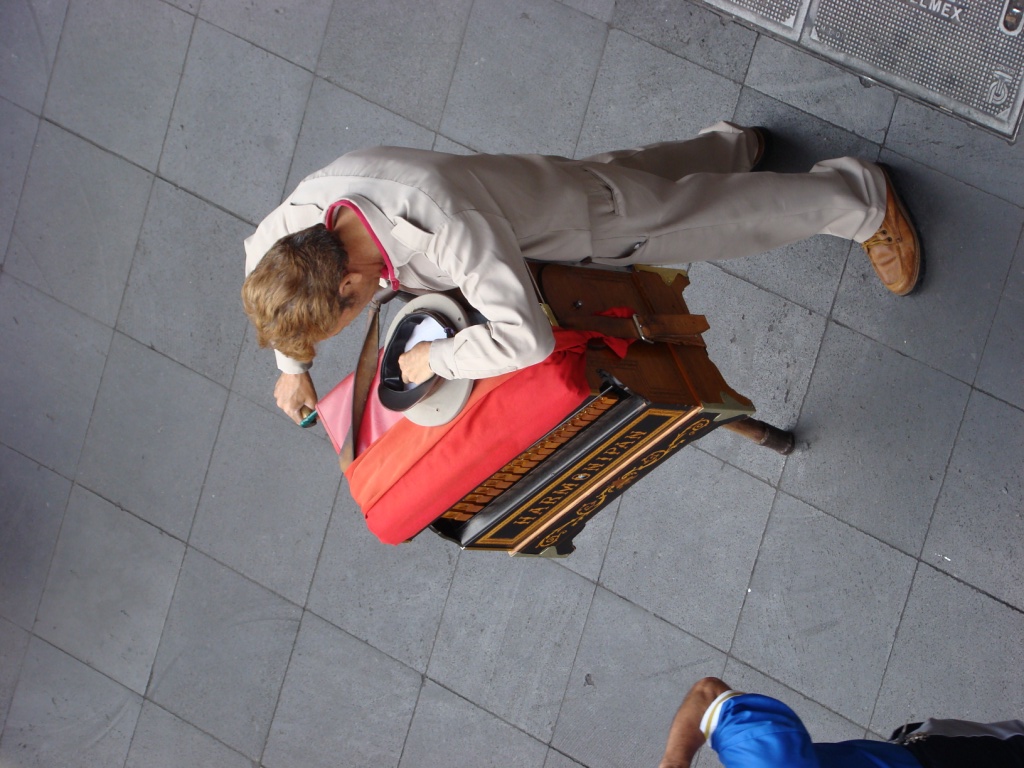The image, taken horizontally but meant to be viewed vertically, captures a detailed outdoor scene. At its center stands a man clad in a light beige uniform, possibly with epaulets, indicating a formal or military style. His uniform includes white pants and brown shoes. The man stands in front of a Harmanipan, a musical instrument or music box with gold lettering on its front and ornate gold details along its brown borders and legs. A red drape, almost like a pillow, adorns the top of the Harmanipan, upon which rests the man's officer-like beige hat. His left hand is placed on the hat, while his right hand operates a lever or handle on the side of the instrument, suggesting he is winding it. Adjacent to him, on the right side of the photo, is another person, identifiable only by their arm and blue shirt. The scene is anchored by a grey stone floor, typical of an outdoor setting, adding to the timeless, evocative atmosphere of the photograph.